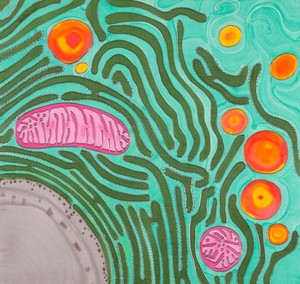This detailed image portrays what appears to be a highly magnified, artistic depiction of a cell. The background is a striking lime green or teal hue, with various darker green lines resembling worms scattered throughout. These dark green, evergreen-like lines become thicker and converge towards the bottom left of the image. At this location, there's a partial view of a large circle with a grayish hue, potentially representing the cell's nucleus. 

Throughout the image, particularly noticeable in the top left and extending towards the right, are numerous circular objects in shades of orange and yellow, resembling cellular components or organelles. 

Additionally, the image features two distinct pink objects: one centrally located on the left side, which is more capsule-shaped, potentially illustrating a mitochondrion, and another circular one positioned at the bottom right. Nestled within the image's intricate design is a small light brown or reddish item with spots on its edges, adding to the rich tapestry of cellular structures portrayed.